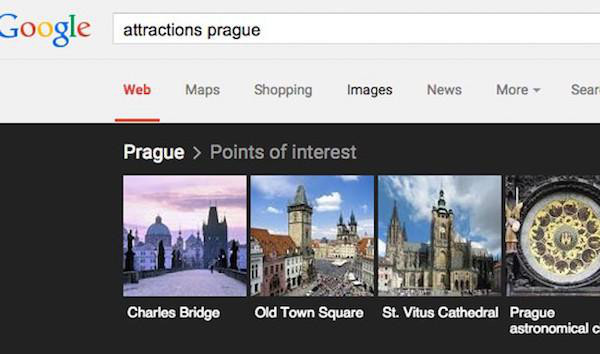A Google web search for "places of interest in Prague" reveals four notable attractions: Charles Bridge, Old Town Square, St. Vitus Cathedral, and the Prague Astronomical Clock. The web page displays a standard search interface with options to refine results by categories such as Maps, Shopping, Images, and News. The highlighted points of interest predominantly feature historical and architectural significance, with images showcasing Prague's iconic older architecture. For instance, the majestic St. Vitus Cathedral, identified by its towering spires, is depicted within the context of the historic Old Town Square, further emphasizing the city's rich cultural heritage.